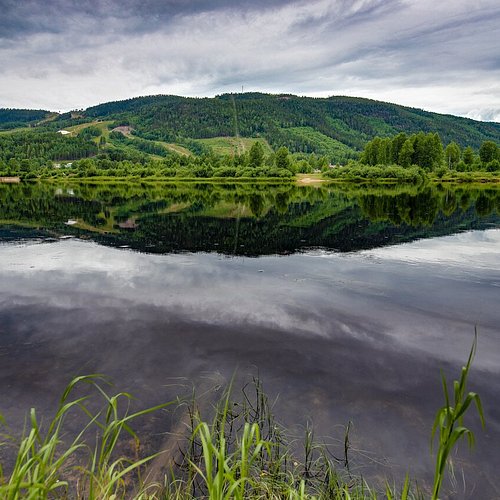This photograph depicts a serene rural setting featuring a lake foreground and a hilly background adorned with dense trees. The middle section of the image showcases a pristine body of water, reflecting both the towering hill and the cloudy sky above. The hill behind the water is predominantly covered in lush, dark green foliage with occasional open areas resembling ski slopes. These open stretches interrupt the greenery, giving the hillside a textured look with sections of flat, mowed ground among the thick forest. 

Closer to the water’s edge, the image captures light green bushes and tall, bright green trees lining the base of the hill. Some small leaves, reeds, and perhaps rocks are visible in the very front of the picture, adding a subtle texture to the immediate foreground. The water itself is highly reflective, mirroring the scattered light gray and dark gray clouds hanging overhead. You can discern a faint hint of a storm either approaching or recently passed, suggested by the dense clouds and the calm, glossy surface of the lake. Off in the distance, blending into the hills, there are a few indistinct buildings or sheds, further enhancing the pastoral atmosphere of this rich and vibrant landscape.